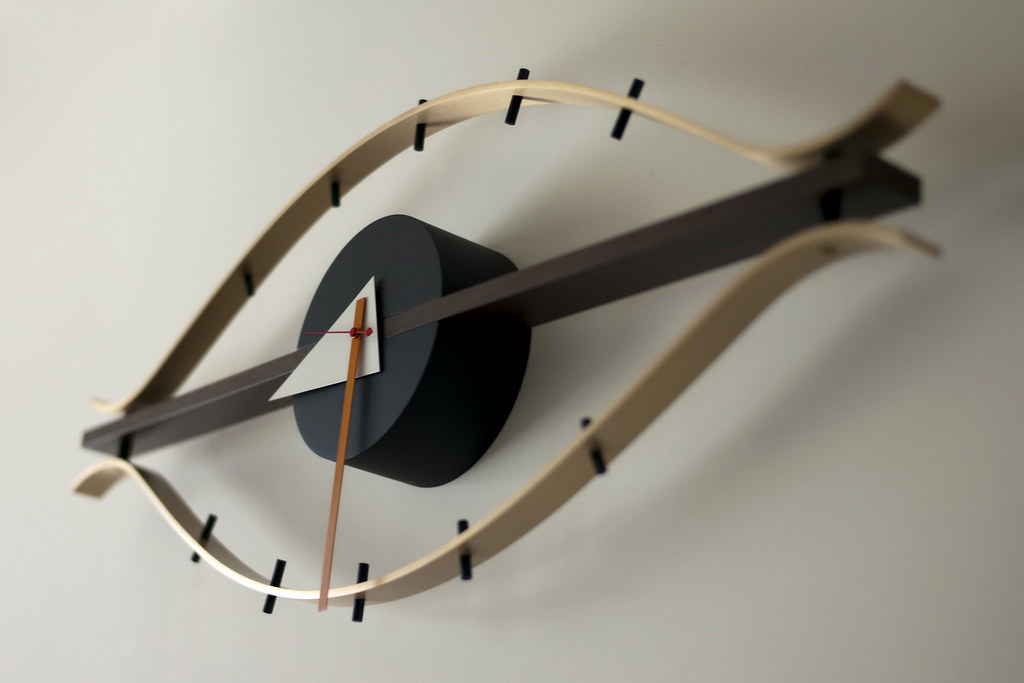This image showcases a unique, eye-shaped Vitra clock mounted on a beige, light tan wall. The three-dimensional clock is designed to resemble a stylized eye. The central feature is a black, round shape akin to a pupil, which protrudes slightly from the wall. A dark brown bar bisects this circle horizontally, extending to the edges of the eye. On either side of this bar, golden metal arcs create the upper and lower curves of the eye, with five symmetrical peg-like protrusions that mimic eyelashes above and below. These eyelashes are beige in color, seamlessly blending with the wall. The minute hand is a silver triangle, the hour hand is a skinny orange line, and the second hand is a thin red line, adding a touch of vibrant color to the clock’s face. This clock, displaying the time as approximately 8:32, combines artistic design with functionality, making it a striking decorative piece.